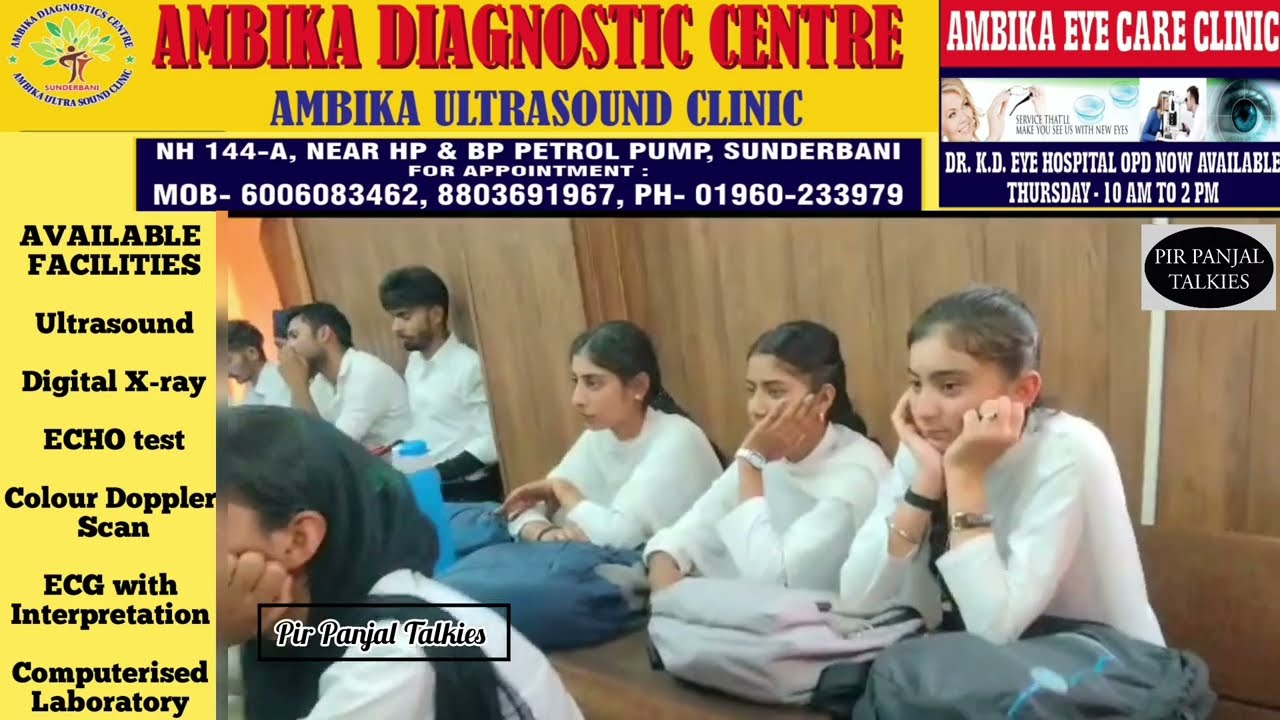This image is a detailed advertisement for the Ambika Diagnostic Center and Ambika Ultrasound Clinic, prominently displayed in bold red and blue text at the top against a yellow background. The ad highlights the clinic's location at NH144-A, near HP and BP petrol pumps, and provides multiple contact numbers for appointments: 600-6083-462 and 880-369-1967 for mobile, and 01960-233-979 for phone. The facilities offered include ultrasound, digital X-ray, echo tests, color doppler scans, ECG with interpretation, and computerized laboratory tests.

To the right, there is additional information about the Ambika Eye Care Clinic, specifying that Dr. KD's Eye Hospital OPD is now available on Thursdays from 10 a.m. to 2 p.m. Below this, a blue box details the location further. The bottom right corner of the image features a section labeled "Peer Pangel Talkies."

In the main image, several individuals, both men and women, dressed in white long-sleeved shirts, are seated on wooden benches against a wooden wall. Some are adorned with bracelets or wristwatches, and they appear to be paying attention to a lecture or presentation.